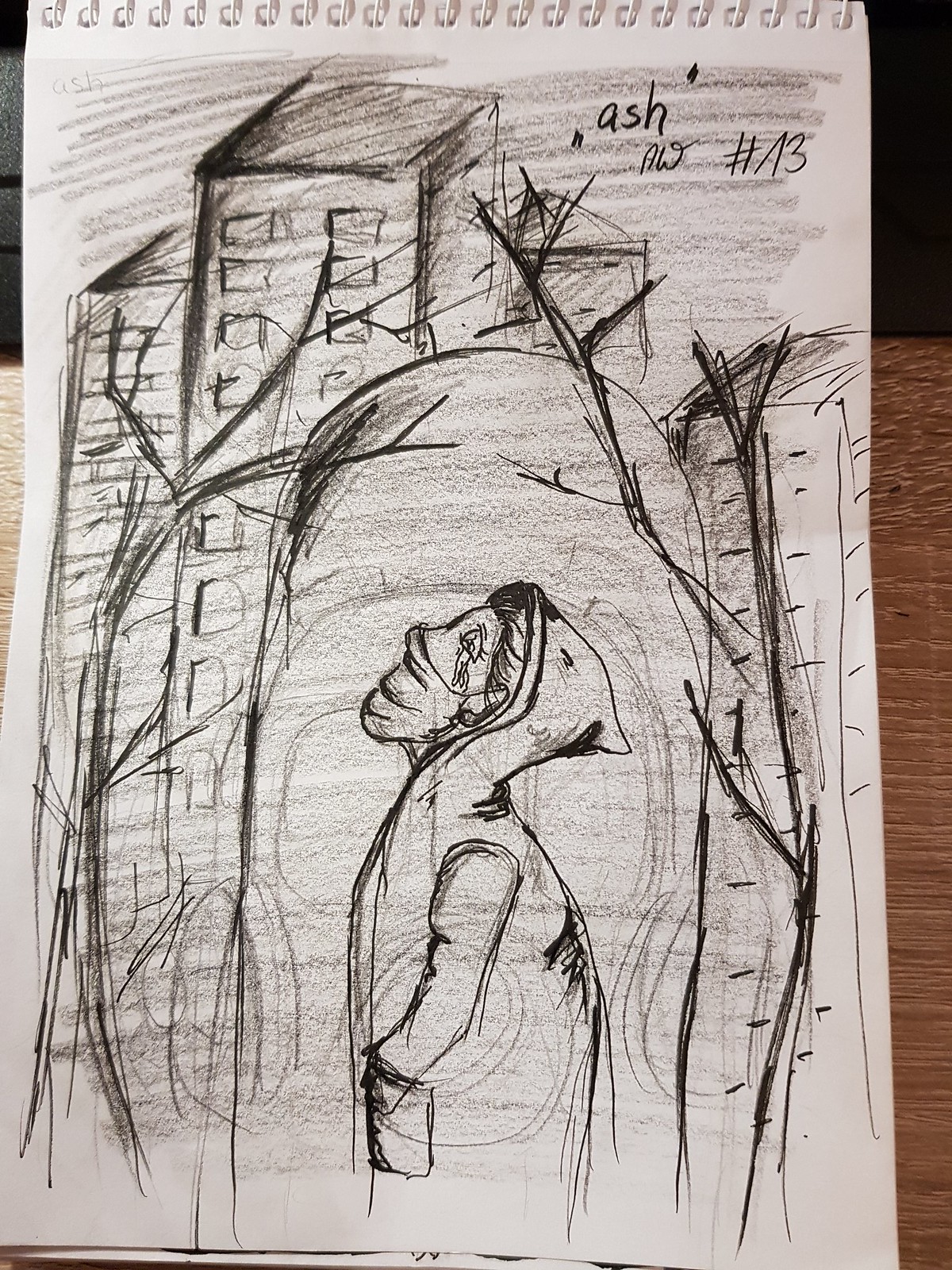This meticulously rendered pencil drawing on a white spiral-bound notebook showcases an urban scene in a portrait orientation. Four buildings dominate the composition, each adorned with detailed windows, capturing an austere cityscape. Amongst the buildings, a few barren trees with intricate branches stand starkly against the monochrome background, devoid of leaves. At the bottom of the image, a solitary figure is depicted wearing a jacket with a hoodie and a COVID-19 style mask. Despite the obscured face, the visible, tear-streaked eye conveys a poignant sense of sorrow. Intriguingly, the upper right corner of the artwork features the inscription "Ash," followed by "A-W," a pound sign (#), and the number 13.